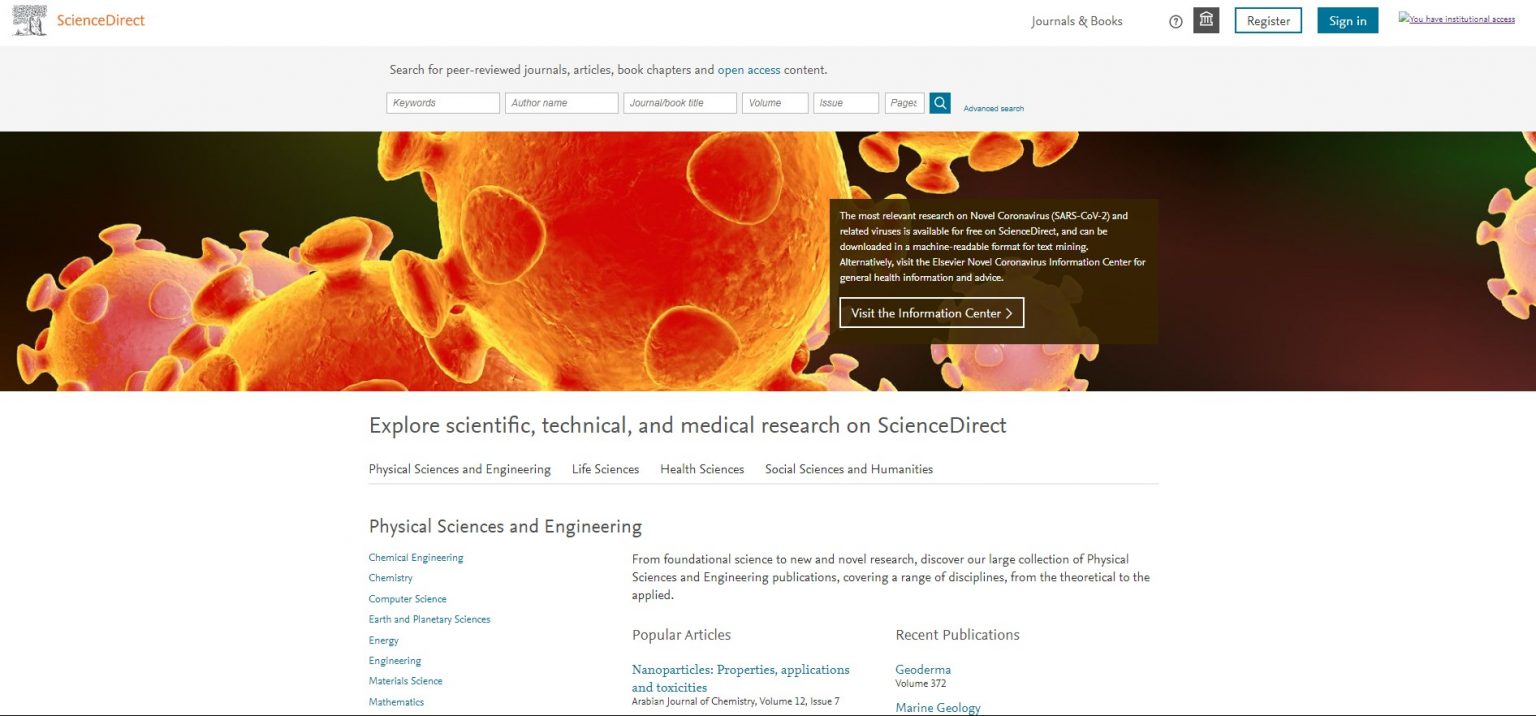The image is a detailed webpage layout for the ScienceDirect website. 

In the top left corner, there's a distinct logo: an icon followed by the brand name "ScienceDirect" in yellow, with an uppercase 'S' and 'D'. To the right of the logo are some interactive elements typical of a site header. First, a white box with a turquoise outline and black text that presumably reads "Register," though it's unclear. Next to it is a solid turquoise button with white text that says "Sign In," followed by additional smaller text elements.

The main section of the page has an off-white background. At the top-center, albeit slightly to the left, there's a small black-font line that starts with "Search for your," followed by text too small to discern. Two turquoise words end this line. Below this header, there are six input boxes aligned horizontally, followed by a turquoise box containing a white magnifying glass icon.

Underneath, there's a large, horizontally-oriented image featuring a series of orange, spherical objects with suction cups. The placement is as follows: one partially visible on the extreme left edge, another half-visible just right of that, a larger one dominating the middle but cropped at both the top and bottom edges, and smaller fragments of others peeking from the right edge. 

Overlaying this image on the right side is a black pop-up box with unreadable white text. The box has a rectangular, horizontal section at the bottom, with white text that reads "Visit the Information Center" followed by a right-pointing arrow (►). Below this segment, in black text, it says, "Explore scientific, technical, and medical research on ScienceDirect," followed by tiny black text, "physical sciences and engineering."

Directly underneath, there's a turquoise-font column aligned towards the left but not entirely left-centered. Adjacent to the right, two more columns contain black-font headings: the first titled "Popular Articles" lists one item in turquoise and black text, and the second titled "Recent Publications" follows the same format. The page concludes with a thin, bolded black line that forms the bottom border.